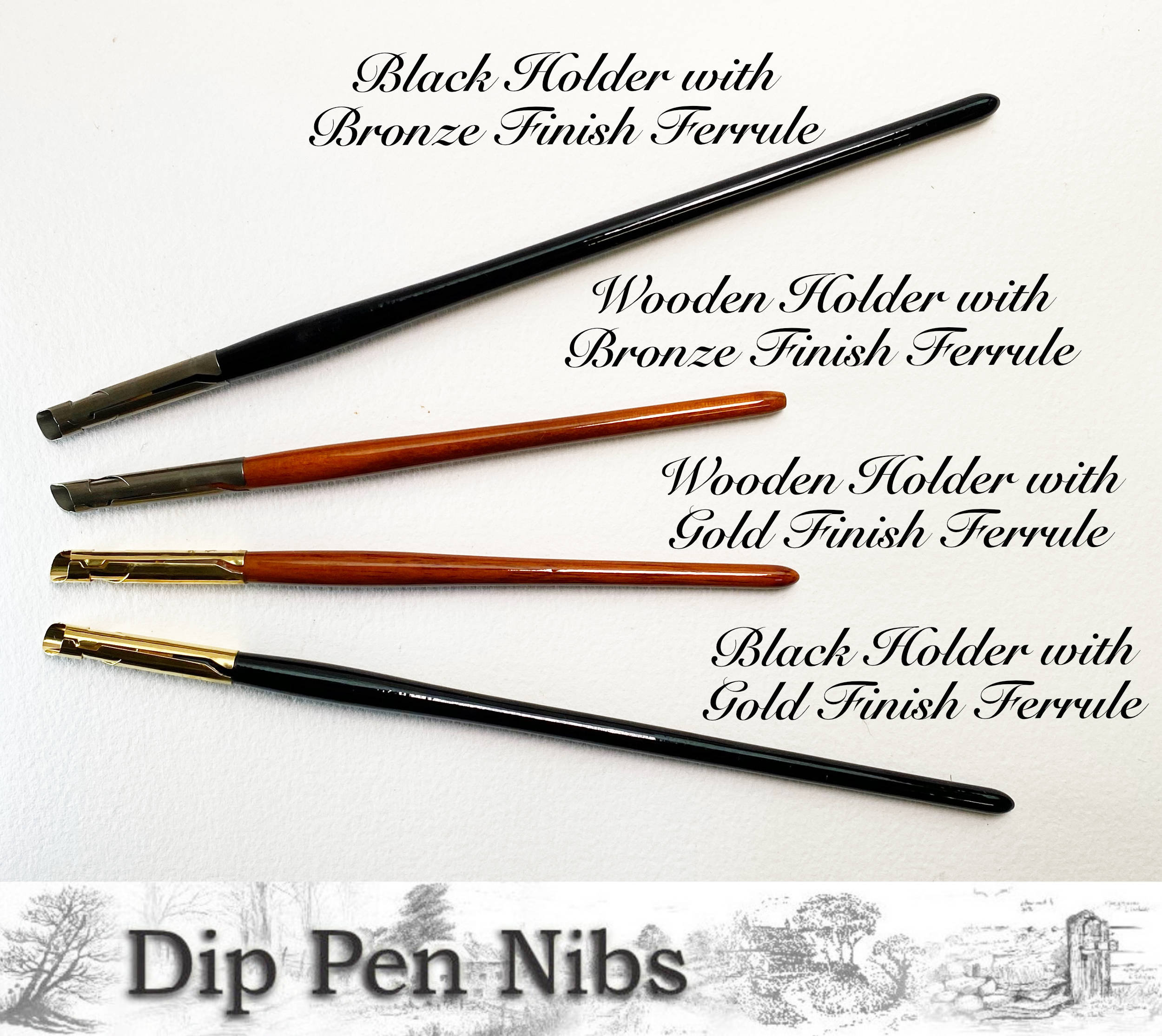This image features what appears to be an advertisement for dip pen nib holders, showcasing four distinct models with detailed descriptions. The holders are arranged on a plain white background. There are two long holders, both black, one with a gold finish ferrule and the other with a tarnished bronze finish. Additionally, there are two shorter wooden holders: one has a bronze finish ferrule, and the other has a gold finish ferrule. While the black holders are sleek and elongated, the wooden ones offer a more compact design. Despite the variations in material and finish, all holders serve the same functional purpose, highlighted by their descriptions which distinguish the gold and bronze ferrule options.